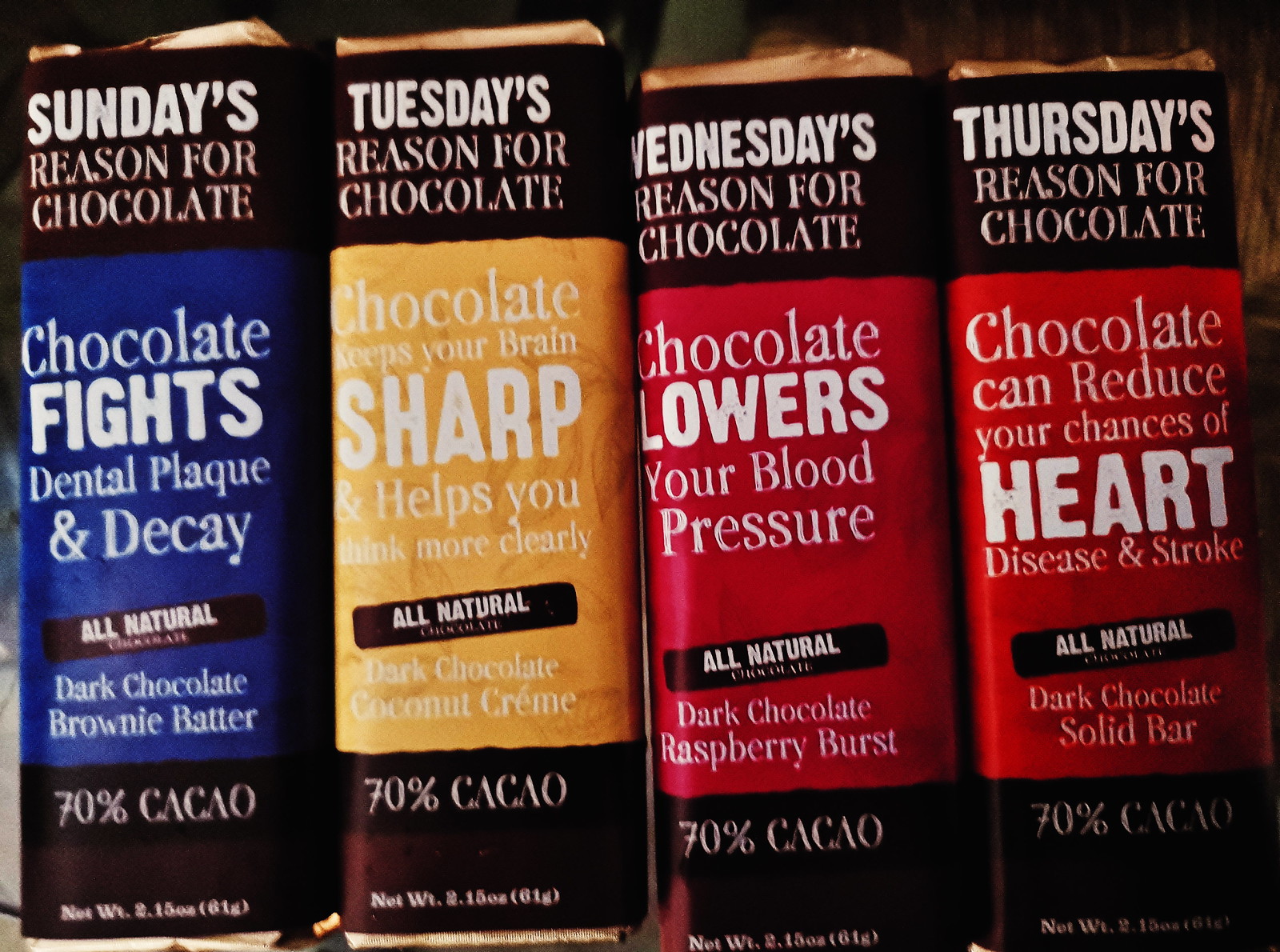The image depicts four different chocolate bars, each detailed with a specific day of the week and a corresponding reason for enjoying chocolate. The bars are presented in distinct, colorful wrappers: blue for Sunday, yellow for Tuesday, red for Wednesday, and orange for Thursday. Each bar contains 70% cacao, weighs 2.15 ounces (61 grams), and is further enclosed in gold foil wrapping. Sunday's blue-wrapped bar reasons that chocolate fights dental plaque and decay with its all-natural dark chocolate brownie batter. Tuesday's yellow-wrapped bar states that chocolate can sharpen thoughts, featuring a dark chocolate coconut cream. Wednesday's red-wrapped bar highlights that chocolate lowers blood pressure and offers a dark chocolate raspberry burst. Finally, Thursday's orange-wrapped bar notes that chocolate can reduce the risk of heart disease and stroke with a dark chocolate solid bar. Despite the image being blurry, the gold accents at the top and bottom of each wrapper add a touch of elegance, while the central colored sections clearly convey the health benefits associated with each day.